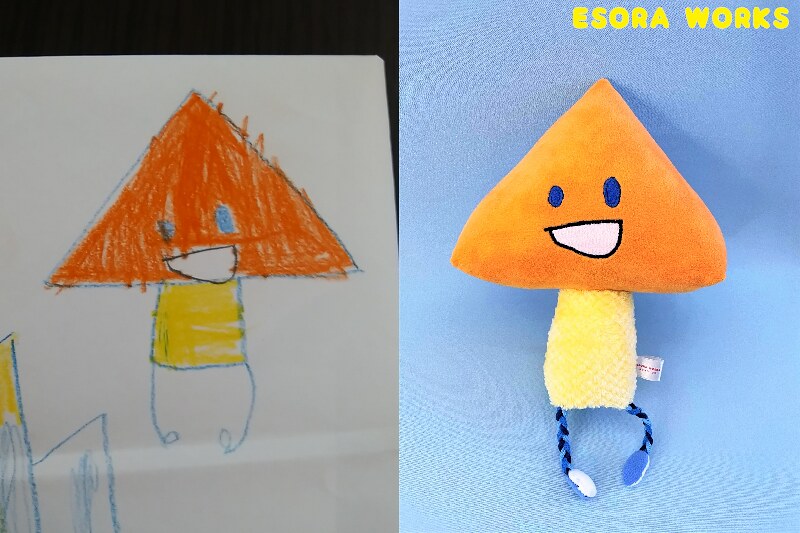This horizontal image features two distinct elements. On the right side, in the upper right corner, there is a plush toy brandishing the label "Isora Works" in yellow text. The toy itself has an orange, triangular mushroom-shaped head adorned with a quirky face; it has asymmetrical blue eyes and a semicircular mouth outlined in black with a white interior. The toy's body is a yellow rectangle, to which blue and black fabric legs—resembling thin shoelaces—are attached. These legs culminate in blue and white shoes. Additionally, there's a yellow tag affixed to the body of the toy.

On the left side of the image, there's a crayon drawing on white paper that depicts this very toy. The artwork captures the toy's unique features with admirable detail and accuracy, showcasing the same triangular orange head, blue eyes, semicircular mouth, yellow rectangular body, and the intertwined blue and black legs with blue and white shoes.